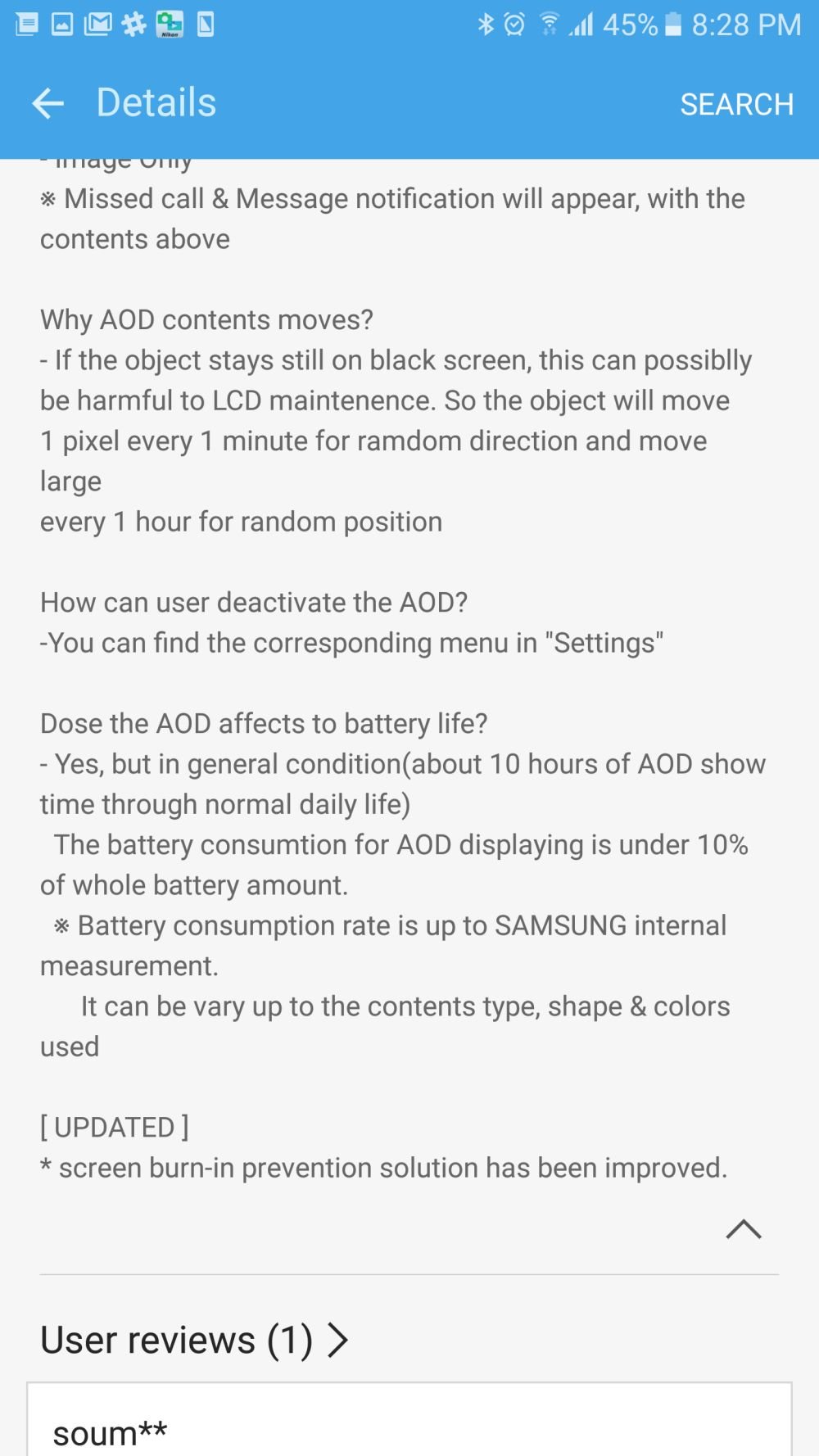The image features a blue bar at the top with a left-pointing arrow next to the word "Details." To the right, it shows the battery life at 45% and the time as 8:28 PM. Below this, an uppercase "SEARCH" option is displayed. 

Centered beneath this, in a large light gray area, several lines of gray text indicate where missed call and message notifications will appear. 

Approximately an inch or two further down, there is a heading: "Why AOD Contents Move." Below this, another heading reads, "How Can Users Deactivate the AOD?" followed by this explanation: "You can find the corresponding menu in 'Settings'."

Another subcategory titled "Does the AOD Affect Battery Life?" includes several lines of informative answers. 

About two inches down, inside parentheses, is the word "Updated," followed by a small asterisk. The text beneath this states that "Screen burn-in prevention solution has been improved."

Finally, at the bottom, there's a section for "User Reviews" with the number "1" in parentheses and an arrow pointing to the right.